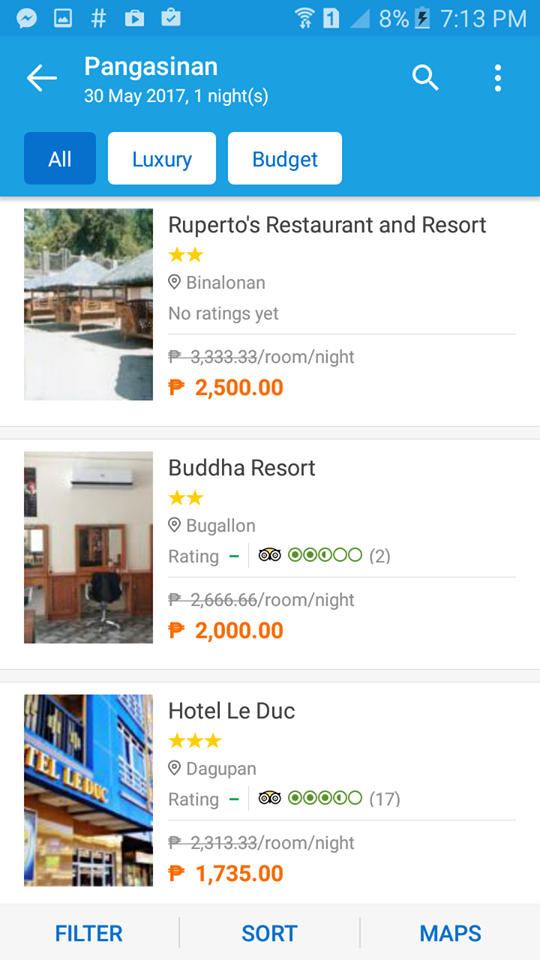The image features a smartphone screenshot with a predominantly white background. The phone's battery is at 8% and currently charging, with the time displayed at 7:13 PM. At the top, there is a back arrow icon to the left, followed by the date "30 May 2017". Parentheses enclose the letter "s". Additionally, there is a magnifying glass icon, representative of a search function, and three vertical dots indicating more options.

Below this, there is a blue rectangle containing the text "All Luxury and Budget" and "All" in white font. 

The main content is set against a white rectangle background and lists different resorts with their ratings, prices, and discount details:

1. **Ruperto's Restaurant and Resort** - Rated 2 stars, initially priced between 2,500 - 3,333.33 pesos per room per night, with prices crossed out.

2. **Buddha Resort** - Rated 2 stars, originally priced at 2,666.66 pesos per room per night, with the price crossed out.

3. **Hotel Lead** - Rated 3 stars, with the initial price listed as 2,313.33 pesos per room per night, also crossed out. 

The crossed-out prices suggest that there might be a discount or new price being offered.